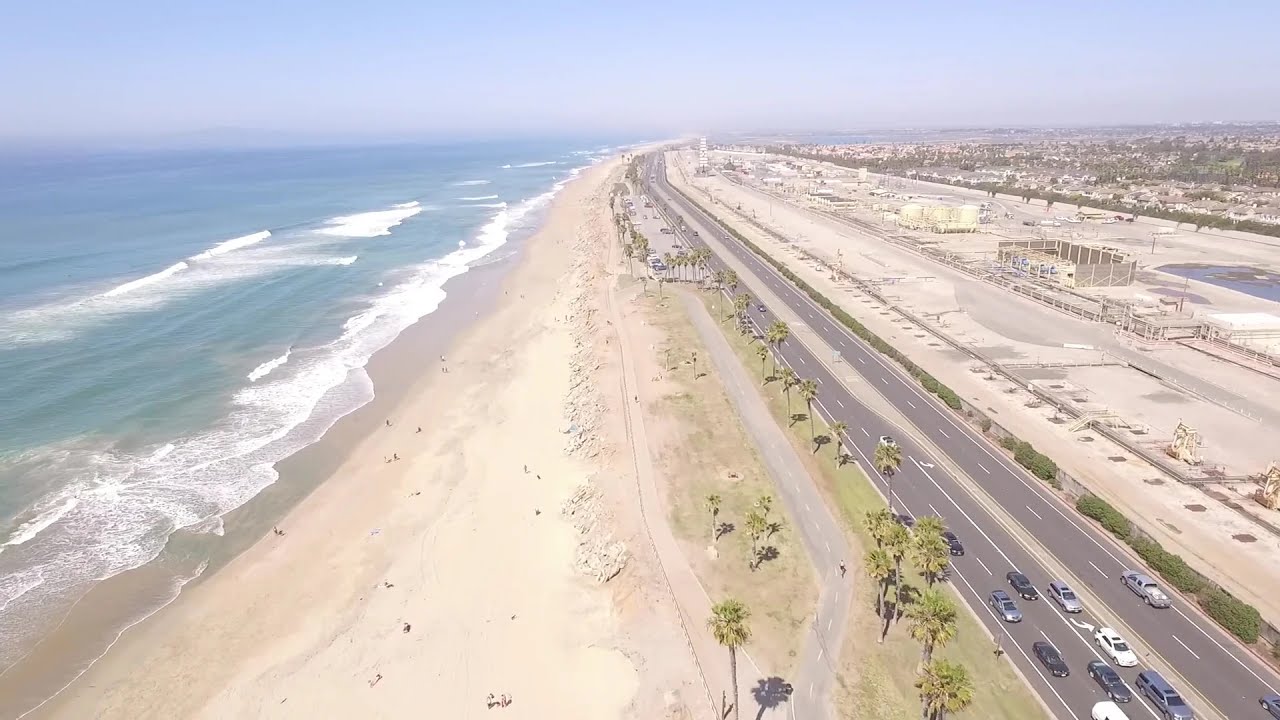This aerial or drone image captures a vibrant coastal scene. To the left, the turquoise-colored ocean laps gently against the shoreline, creating a stretch of white water and small waves that blend into the sandy beach. The beach is adorned with sparse palm trees and features a well-maintained pedestrian path. A two-way highway with three lanes on each side runs parallel to the beach, with about eight cars traveling in one direction, heading towards the back of the image. 

On the right side of the highway, the landscape transitions into an industrial area marked by asphalt, machinery, metal structures, and tanks, all sparsely distributed across the sandy terrain. Further to the right, there are buildings under construction and a suburban residential zone with similar-looking homes, suggesting it might be a planned community. This area is surrounded by more greenery.

The sky above is overcast and hazy, giving the scene a diffused, softened daylight. Given the style of buildings and types of cars, this image could be of a coastal region in North America or a similar beach location elsewhere.